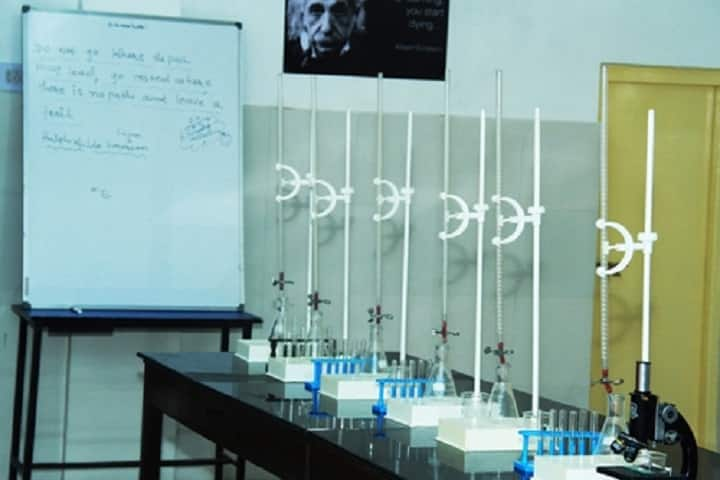The image depicts a detailed and well-equipped science or chemistry classroom. Dominating the room is a long, rectangular black table with an assortment of scientific instruments and equipment arranged neatly on top. Among these instruments are microscopes, blue vial holders filled with test tubes, and several beakers. Each of the six stations also features various test tubes and beakers, with tall white poles or stands that seem to be used for supporting filters or funnels leading into the beakers. Interspersed among the apparatuses are trays with green bottoms and white tops, which hold different materials.

Behind the table, the wall is painted green and prominently displays a striking portrait of Albert Einstein set against a black background. To the left of this poster, a whiteboard filled with written text is mounted, contrasting with the green wall. Moving to the right side of the room, there is a vibrant yellow door with a black handle. The layout and specific details, like the color-coded test tube holders and the arrangement of equipment, underline the organized and practical nature of the classroom setting.